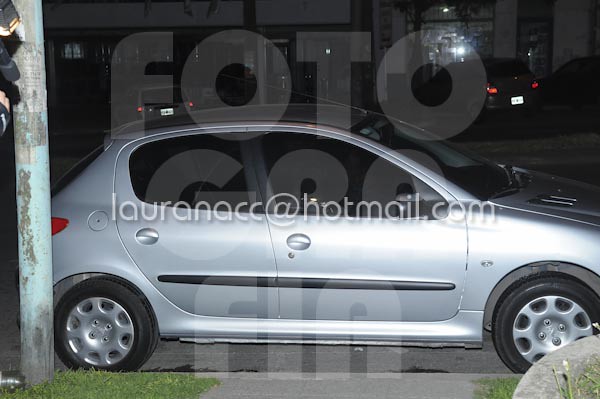This nighttime photo showcases a compact four-door car that resembles a Honda Civic, though somewhat smaller. The vehicle is parked curbside, aligning with a sidewalk that appears slightly blocked by its presence. The car's color is a light blue-silver, and it features black wheels with gray hubcaps. The windows are entirely blacked out, making the interior invisible. In the background, another vehicle is seen, its rear lights illuminated, along with faint outlines of buildings. A slightly rusted blue traffic pole stands next to the car, contributing to the urban scene. There is a clear sidewalk with patches of grass around it. The image contains faint watermarks; one reads "photo" followed by indistinguishable characters, potentially "CRA" or "GRA," and "FIA." Prominently, the email "LauraNACC at hotmail.com" is displayed in white text across the center of the image.